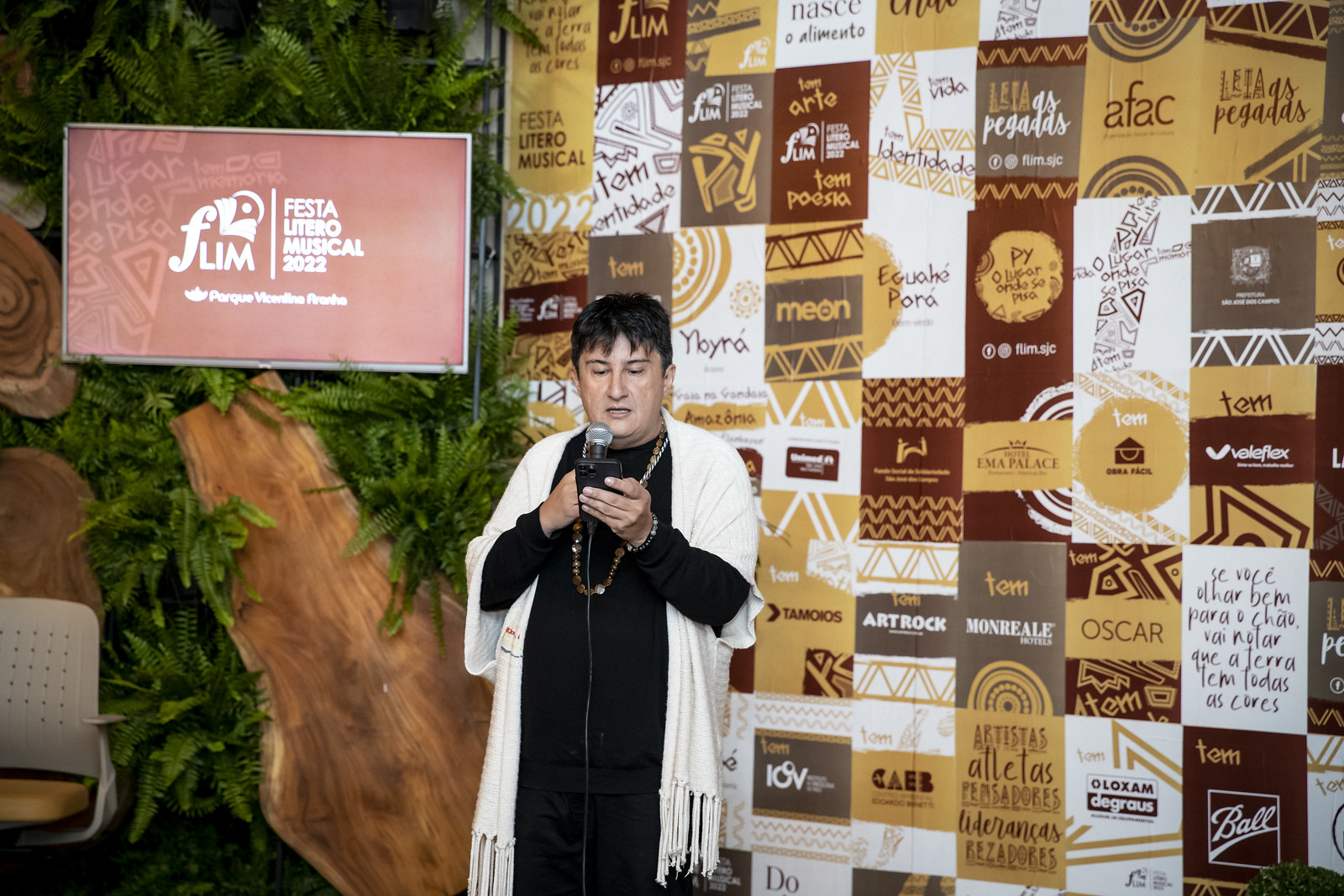This image features a serious-looking individual, likely a religious figure, standing centrally and facing the viewer. The person is dressed in a black top and pants, adorned with a cream-colored, short-sleeved vest with tassels. They have short black hair, dark eyebrows, and wear a gold chain or necklace. In their left hand, they hold a phone, while a wired microphone with a silver head is in their right hand. 

The background is a mosaic-like wall filled with rectangular and square posters in shades of mustard, rust, and white, predominantly in a language other than English. Notable texts include "Oscar," "A-F-A-C," and "Festa Litero Musical 2022." Additional posters carry similar thematic colors and advertisements, pointing to a cultural or musical event.

To the individual's left (viewer’s right) are wooden slabs, a tan chair, and lush green ferns. Among the ferns, a poster displaying "Festa Litero Musical 2022" is visible, maintaining the consistent color scheme of the backdrop. The scene is both vibrant and intricate, enriched with cultural references and detailed advertisements, suggesting an event of significant importance.